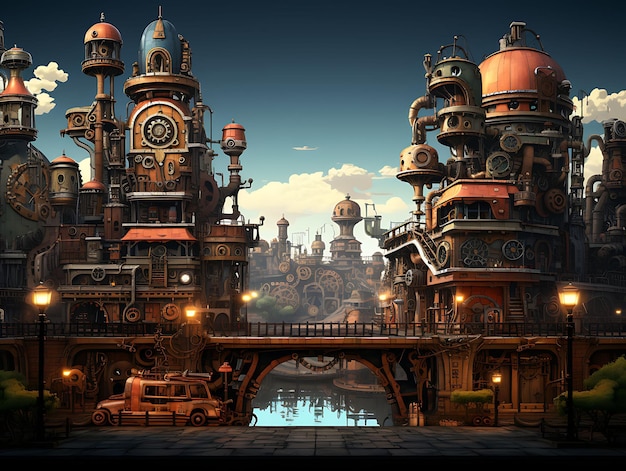The image portrays a highly detailed, retro-futuristic steampunk cityscape, bursting with whimsical and imaginative features. Dominating the foreground is a cobblestone walkway that leads up to a unique, tractor-taxi hybrid vehicle. Just beyond, a wooden bridge spans a body of water, possibly a river or lake, nestled beneath tall, intricately designed buildings. These structures are adorned with an array of round domes, twisting metal pipes, tunnels, and tubes, with sprockets and gears affixed to the exterior surfaces. 

Multiple levels of architecture create a layered effect, featuring round windows and stairways. Street lights dot the scene sporadically, enhancing the surreal ambiance. In the far background, another massive building stretches across the entire horizon, echoing the same curvilinear and abstract architectural style. Despite the dark sky above, clear blue skies are visible beyond, underscoring the painting's cartoonish and imaginative nature. This vibrant and chaotic depiction captures the essence of a fantastical city in an almost "monster civilization" style, blending steampunk elements with a playful, otherworldly aesthetic.